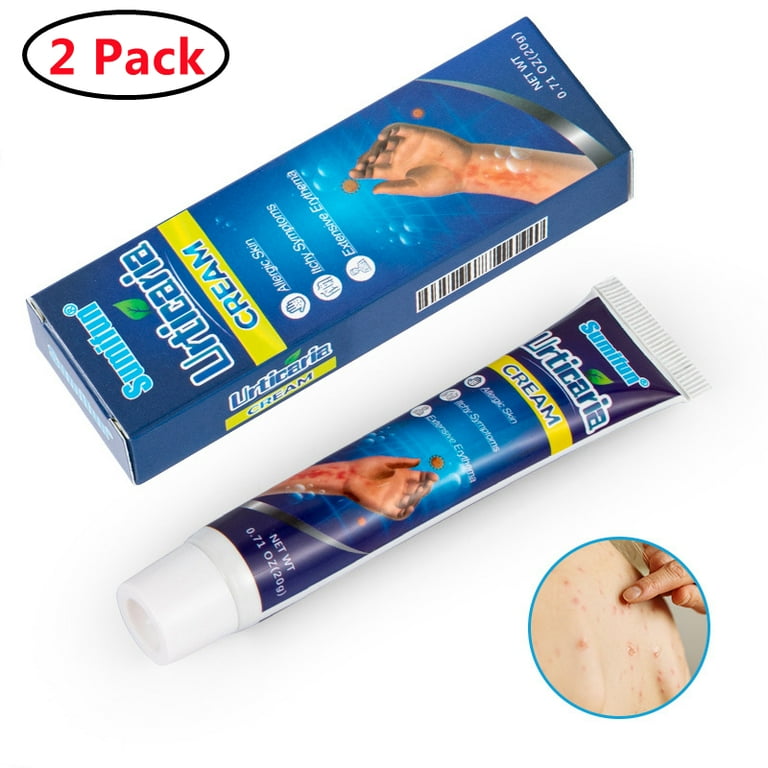This advertisement promotes a 2-pack of Summifun Urticaria Cream, specifically designed for allergic skin, itchy symptoms, and extensive erythema. The top left corner features the text "2-pack" in red letters inside a black oval. Below this, a blue and yellow box displays the product name "Summifun Urticaria Cream," including detailed claims about its effectiveness against allergic skin issues and itchiness. The tube of cream, depicted in both the box illustration and separately below, is white with blue and yellow accents, and contains 0.71 ounces of the cream. Additionally, in the bottom right corner, there's a circular diagram showing a hand pointing to an individual's back, which is covered in red bumps, possibly indicating an allergic reaction or eczema. The design elements, such as the color scheme of blue, yellow, and white, are consistent across the packaging, emphasizing the product's medical efficacy and aesthetic appeal.